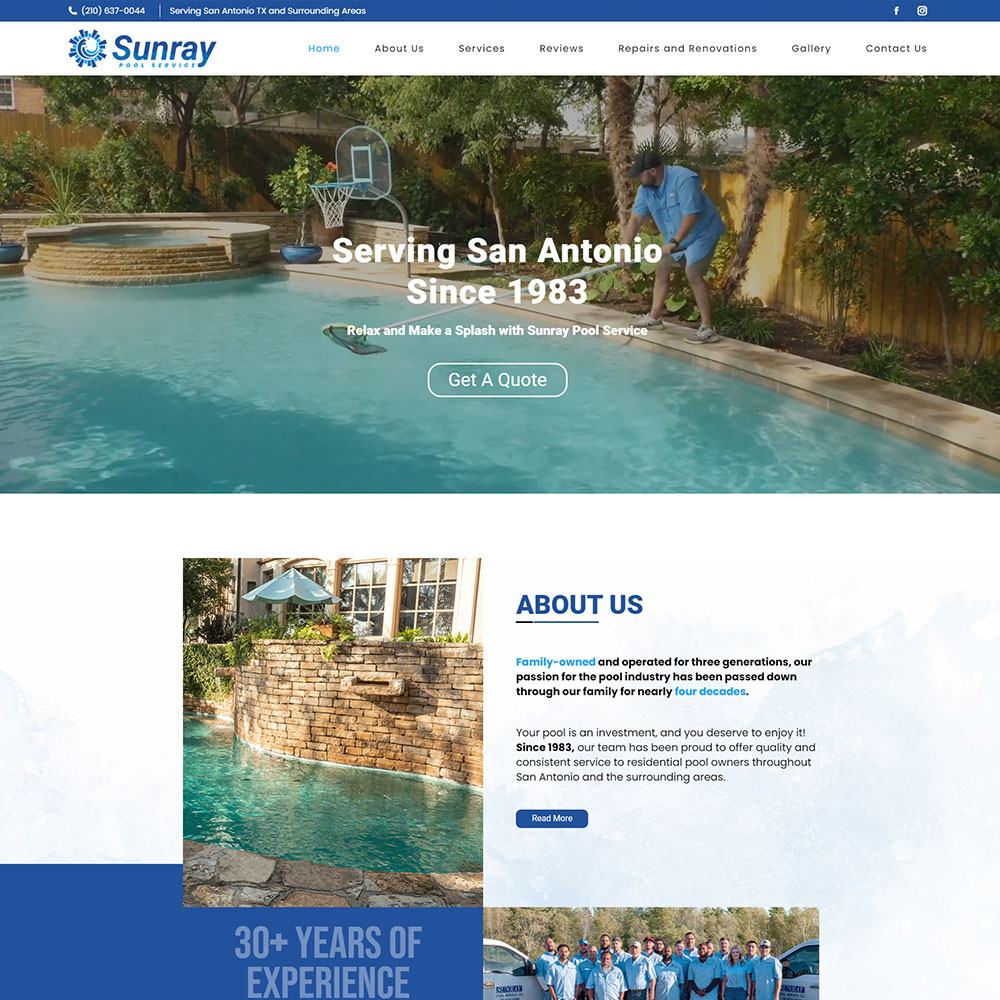The image showcases the homepage of the Sunray Pool Services website. At the top of the page, there is a prominent blue and white banner featuring a phone number for inquiries, along with text indicating that their services extend to San Antonio, Texas, and its surrounding areas. To the upper right corner, Facebook and Instagram icons are visible for social media connections.

Centered on the banner, the Sunray logo appears—a captivating swirl of light blue and navy blue hues. Adjacent to the logo on the right, a navigation menu includes tabs for "Home," "About Us," "Services," "Reviews," "Repairs and Renovations," "Gallery," and "Contact Us."

Below the banner, a vivid image displays a Sunray employee in action, diligently cleaning a pool with a long-handled net. Text alongside the image reads, "Serving San Antonio since 1983. Relax and make a splash with Sunray Pool Services."

Further down, an "About Us" section features a secondary image of a pristine pool and mentions "Three years plus of experience," complemented by a photograph of the dedicated Sunray staff.